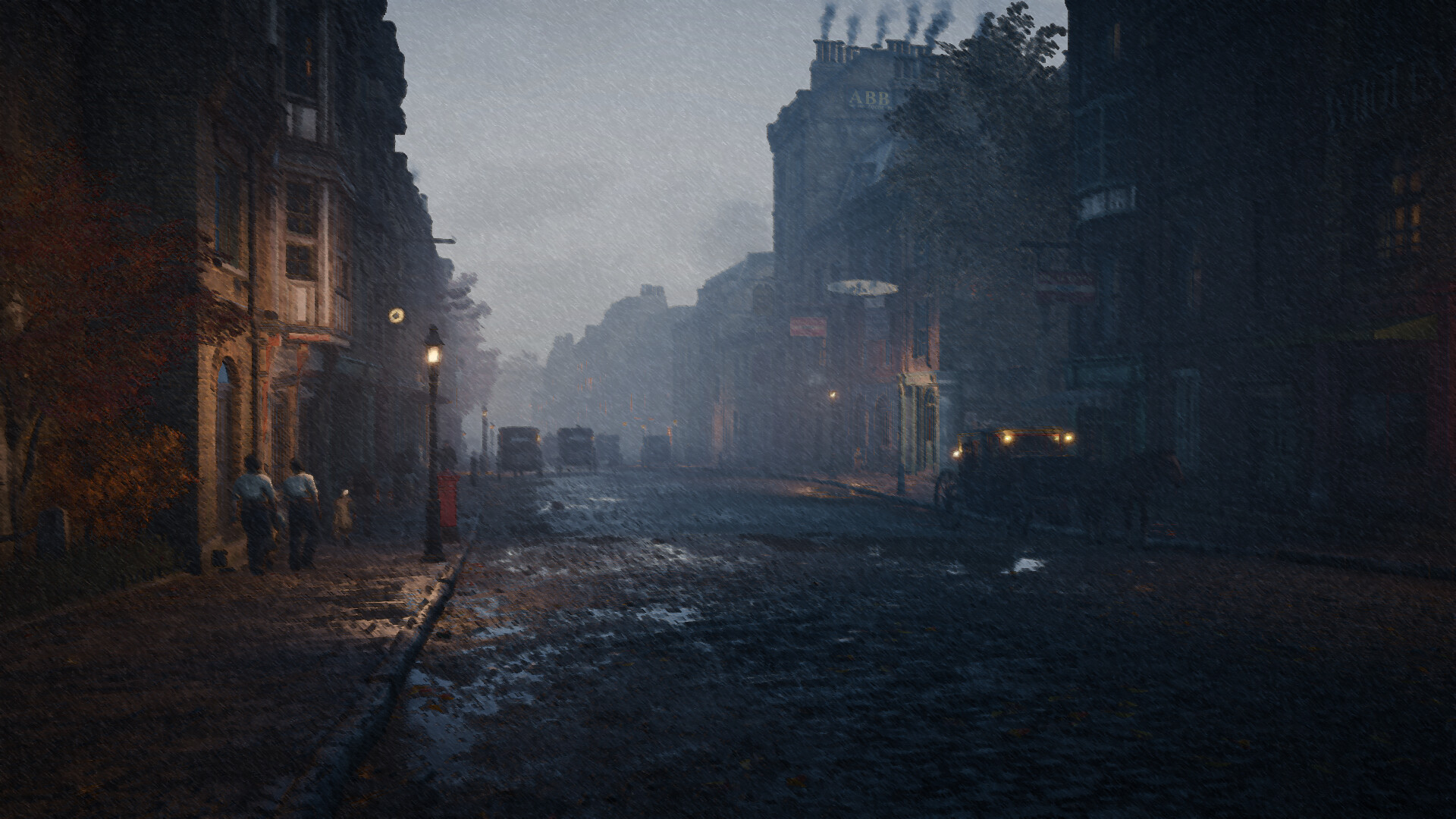The image showcases a gloomy, rain-soaked city street, perhaps reminiscing the 1920s. The perspective is from the middle of the cobblestone street, flanked by multi-story buildings that might be townhouses. The scene is dim and dusky, with a foggy, overcast sky that makes it appear as if it's either dawn or dusk. Old-fashioned street lamps and gas lights line the sidewalks, casting a faint glow on the wet road, creating reflections in the puddles.

On the sidewalk to the left, near the closest building, stand three figures: two individuals in white shirts and a smaller figure, possibly a young girl, in a brown dress. Several cars from the early 20th century, reminiscent of Model A or T Fords, are parked along the street. The right side of the street reveals a more industrial building with five smokestacks emitting smoke, indicating a factory. Nearby, a street lamp illuminates a doorway to some stores, providing a touch of light in the dim setting.

In the distance, further down the road, more vehicles can be seen, their forms blurred but indicative of an older era. The overall scene, though appearing old-fashioned, might be a contemporary artistic depiction, with meticulous details like the wet, muddy dirt road and the subtle lighting techniques enhancing the nostalgic ambiance. The windows of the buildings are mostly dark, hinting at either early morning or evening time, adding to the painting's quiet and contemplative mood.